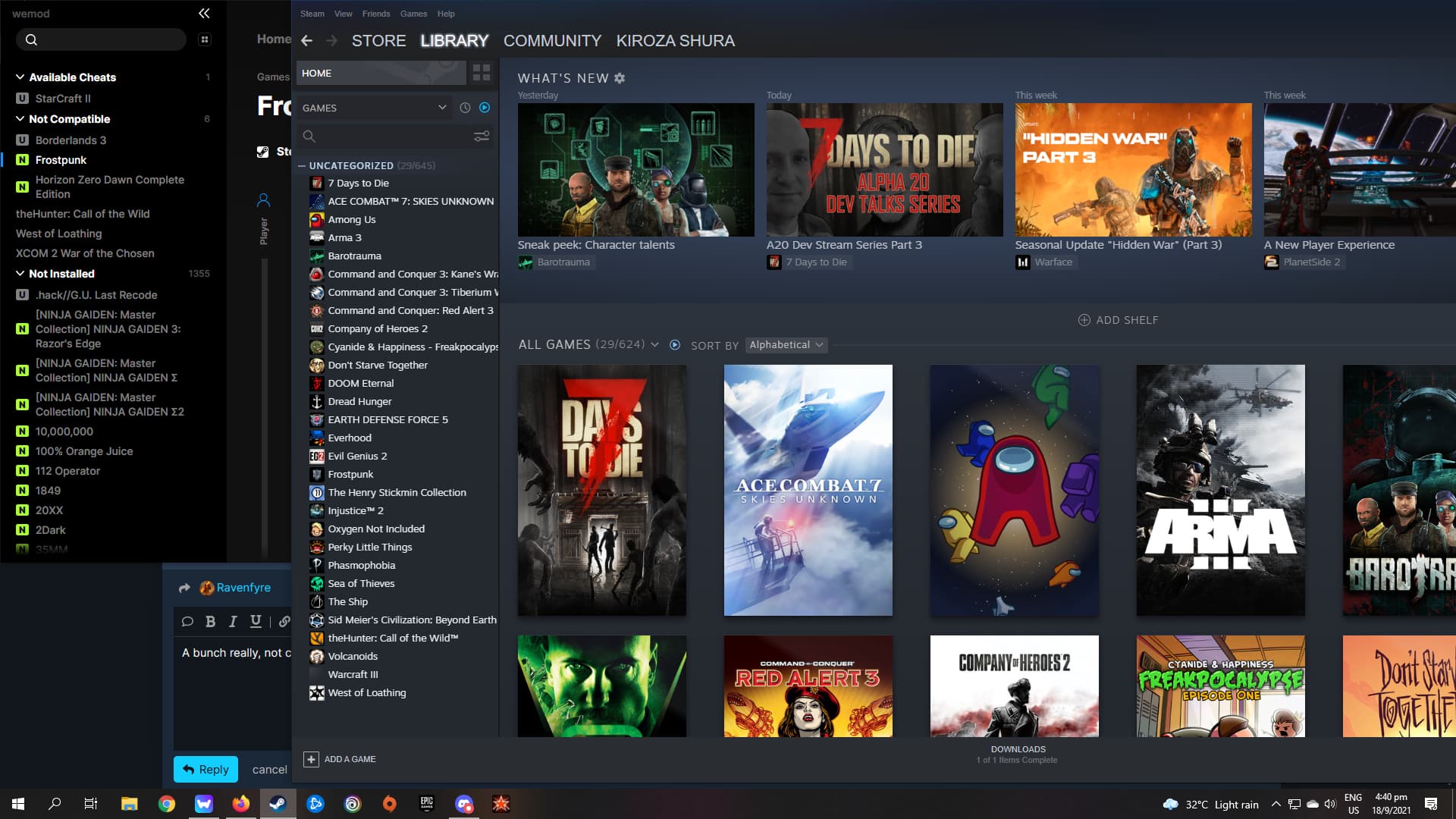Here's a detailed and cleaned-up caption for the described screenshot:

---

**Detailed Screenshot Description:**

The screenshot appears to be from the **Sony PlayStation Store** interface. The top section features a charcoal gray background with white text displaying menu options: **Store, Library, Community, Kuroza Shura**. In the upper left corner, a dark gray bar contains a white search icon. 

A vertical column on the left-hand side of the screen is divided into categories, each bolded in white text, such as **Available Cheats, Not Compatible, Frostpunk, Not Installed**. Game titles listed under these categories have small green square icons with an "N" beside some of them.

A pop-up window in the center reiterates the main menu options (**Store, Library, Community**). Adjacent to this, another vertical column features a search bar at the top labeled **Games**, which is accompanied by a white drop-down arrow and a blue button to the right. Below it, a list of video games is displayed against a black background with bold white text. These games are under the category **Uncategorized** and include titles like **Seven Days to Die, Doom Eternal, Command and Conquer 3, Frostpunk, Real Genius 2, Volcanoids, Warcraft 3,** and **West of Loathing**. At the bottom, there’s a white square icon with a white arrow and a plus sign beside the text **Add a Game**.

On the right side, three rows of horizontal thumbnails display various video games. The first row, titled **What's New**, features four game boxes. The next two rows, under the label **All Games**, show additional thumbnails organized similarly.

To the left of the games list in the central pop-up window, an active text chat window is displayed, with a user named **Ravenfire** highlighted in blue on a gray background. The text chat shows a snippet of conversation: “a bunch really common, not something.” Below this chat, options to **Reply** (blue button) or **Cancel** (white text) are available.

At the bottom of the screen, a Windows taskbar is visible. Icons include the four-pane Windows logo, search icon, file manager, Chrome, WordPad, Firefox, Steam, an unfamiliar blue and white triangle icon, a white circle icon, a red Q, an EPC label in white, the Discord app (with a message notification), and an orange star. In the lower right corner, a white cloud icon indicates the weather as **32°C, light rain**, and the time is shown as **4:40 PM** with the system language set to English.

---

This detailed caption provides a clear and comprehensive overview of the screenshot, highlighting the key elements and structure of the PlayStation Store interface along with contextual information shown on the user's Windows taskbar.